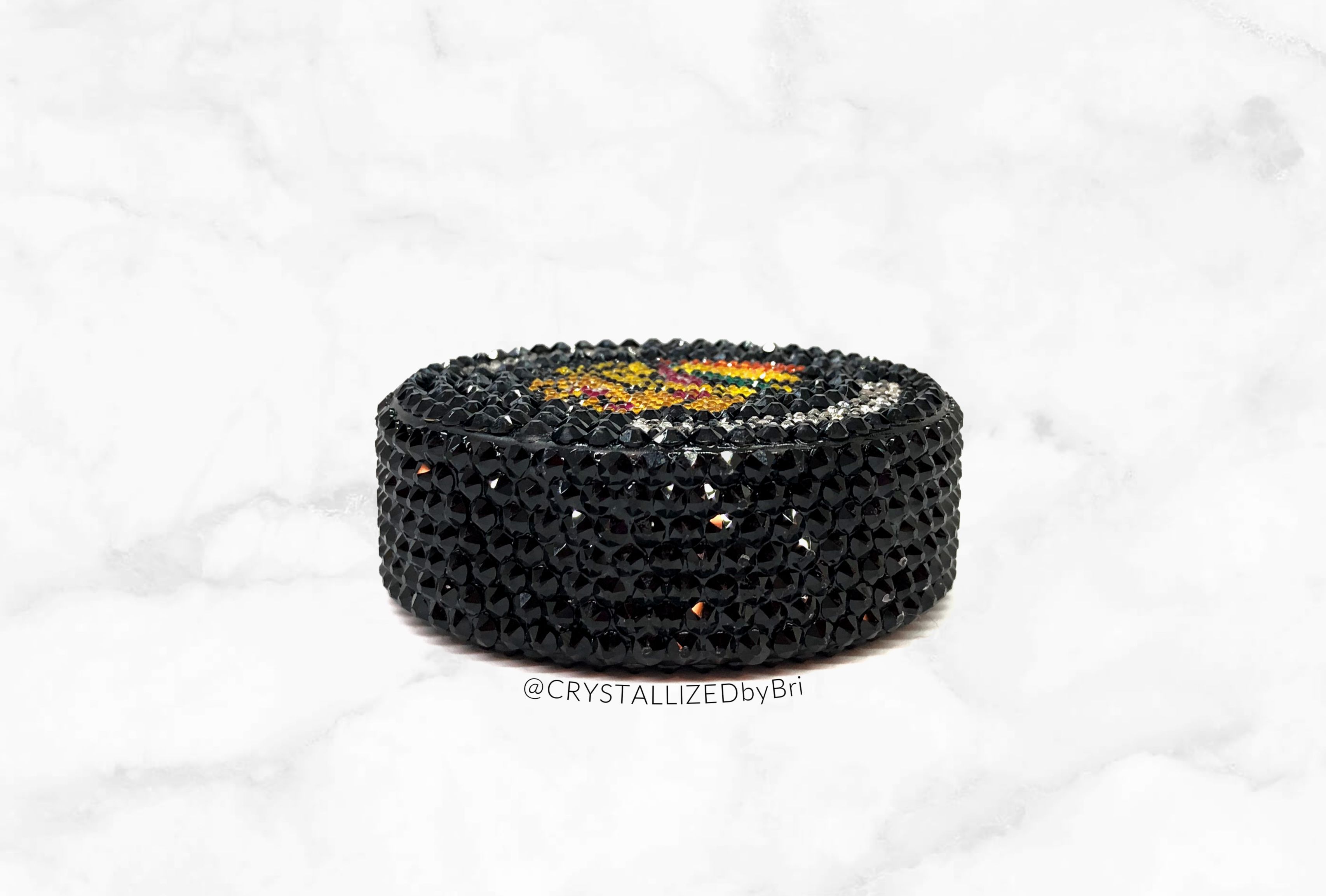The image depicts a black crystal figurine viewed from the side, prominently displaying its intricate details. The figurine, crafted from thousands of black crystals, showcases a textured surface with small divots that create a gleaming sheen. At the top, a semi-circle of white crystals contrasts against the black, and the middle features an intricate design with yellow, red, and green crystals. Perhaps resembling a car wheel or a jewel, the figurine's shape and design elements hint at its artistic complexity. Resting on a white marble background, the piece is titled "Crystallized by Brie," as indicated by the inscription below it.